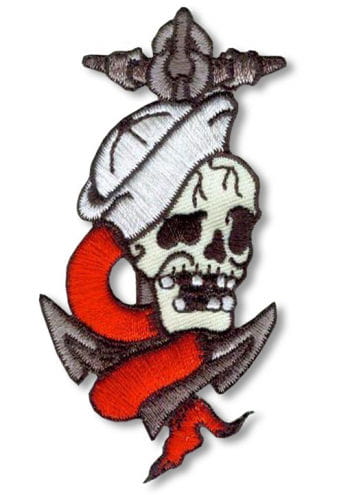The image showcases a detailed embroidery patch designed with a nautical theme. At the forefront is a large, silver-gray anchor, characterized by its traditional shape with a curved bottom and three spikes—two pointing upward and one downward. Prominently featured in front of the anchor is a white skeleton skull, with hollow black eyes and nose cavities. The skull displays a partially open mouth, revealing six teeth with noticeable gaps where teeth are missing, and exhibits two prominent cracks running down its forehead. Adorning the skull is a white sailor hat, which is tilted to the left side. Encircling the anchor and emerging from behind the skull is a red ribbon that wraps intricately around the anchor, ending in a tattered black fashion at the bottom. The patch itself is set against a pure white background, highlighting the intricate details and colors of the design.